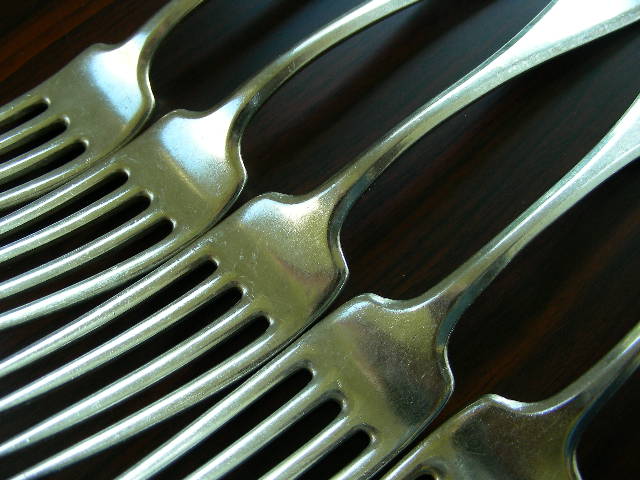This close-up image captures five highly polished forks, either made of silver or stainless steel, arranged diagonally from the upper left to the lower right. The forks, each with four even tines, are laid out on a dark wooden table, with the rich grain clearly visible. The photograph focuses on the transition from the handle to the tines, cutting off parts of the forks, which suggests the artistic intent behind the shot. Reflections on the forks' surfaces reveal a hint of the surrounding dark wood and slight rainbow oxidation, adding depth and detail to the image.